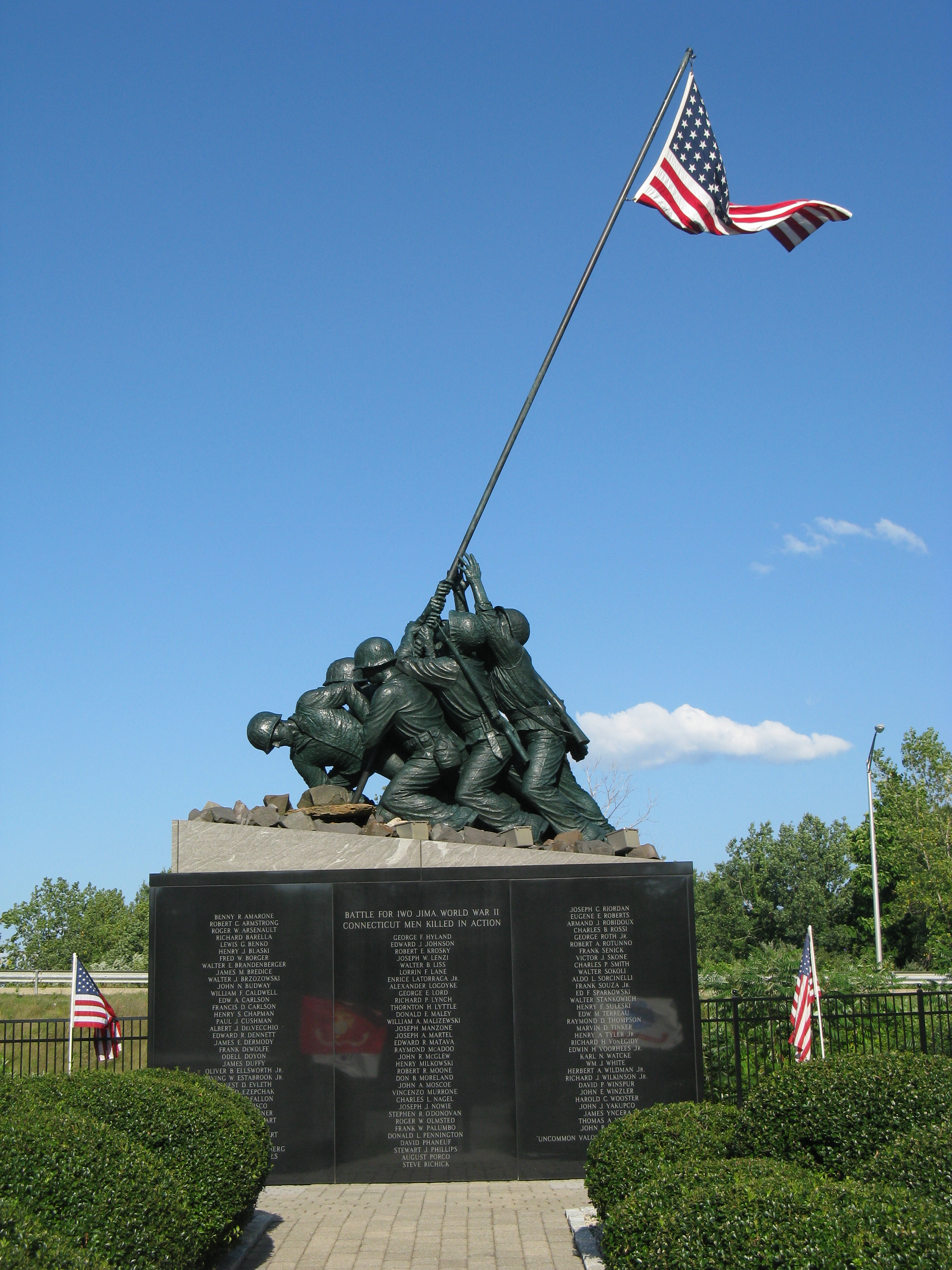This image portrays a detailed and evocative war memorial dedicated to the Battle of Iwo Jima during World War II, specifically honoring the men killed in action. The memorial features a prominent bronze statue of Marines in the iconic pose of raising the American flag, reminiscent of the famous photograph taken during the battle. The figures are depicted straining with effort, with several soldiers on their feet and knees pushing the flagpole into the ground. The flag itself is captured mid-flutter, blowing in the wind against a bright blue sky with a few scattered clouds. 

The memorial stands upon a brown marble base with white engraving, detailing the battle and the heroes from Connecticut who perished. Three black stone panels, inscribed with many names (though illegible from this distance), form the wall below the statue. Flanking the walkway leading up to the memorial are neatly trimmed dark green shrubs, and two smaller American flags on white sticks planted into the ground. The scene is set in a park with additional landscaping, including trees in the background, adding to the serene and respectful ambiance of the site.